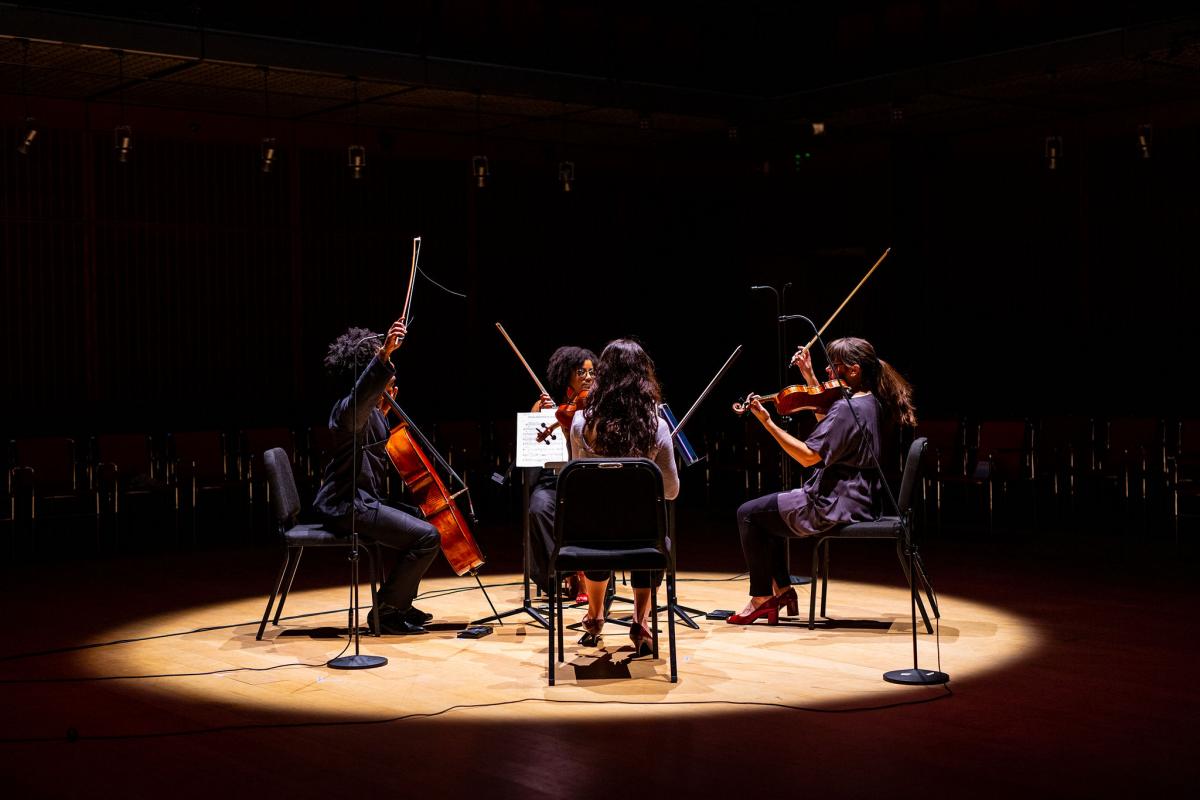In a dimly lit, empty auditorium, four young female musicians sit in a circle under an oblong, bright spotlight. Their metal chairs, with black seats and backs, are positioned in the center of a wooden stage. The spotlight reveals the intense focus and spirited nature of the performers, each dressed in dark purple tunic-length T-shirts and dark pants. The woman closest to the viewer has long, free-flowing hair and wears black pants that end below the knee with black shoes. Her bow is raised, and her music stand stands before her. To her right, another musician, with a violin and high red heels, holds her bow high with her long hair tied back. Across from the first woman, another musician, partially obscured, shows only her leg and head, with black hair, as she turns towards the violinist. The most animated performer to the left, a young woman of color with high, curly hair, handles a cello, her bow raised in her right hand, the cello resting on the ground. Empty metal chairs with wooden backs are visible in the darkened background, along with dim or unlit lights, adding to the atmosphere of a captivating rehearsal.